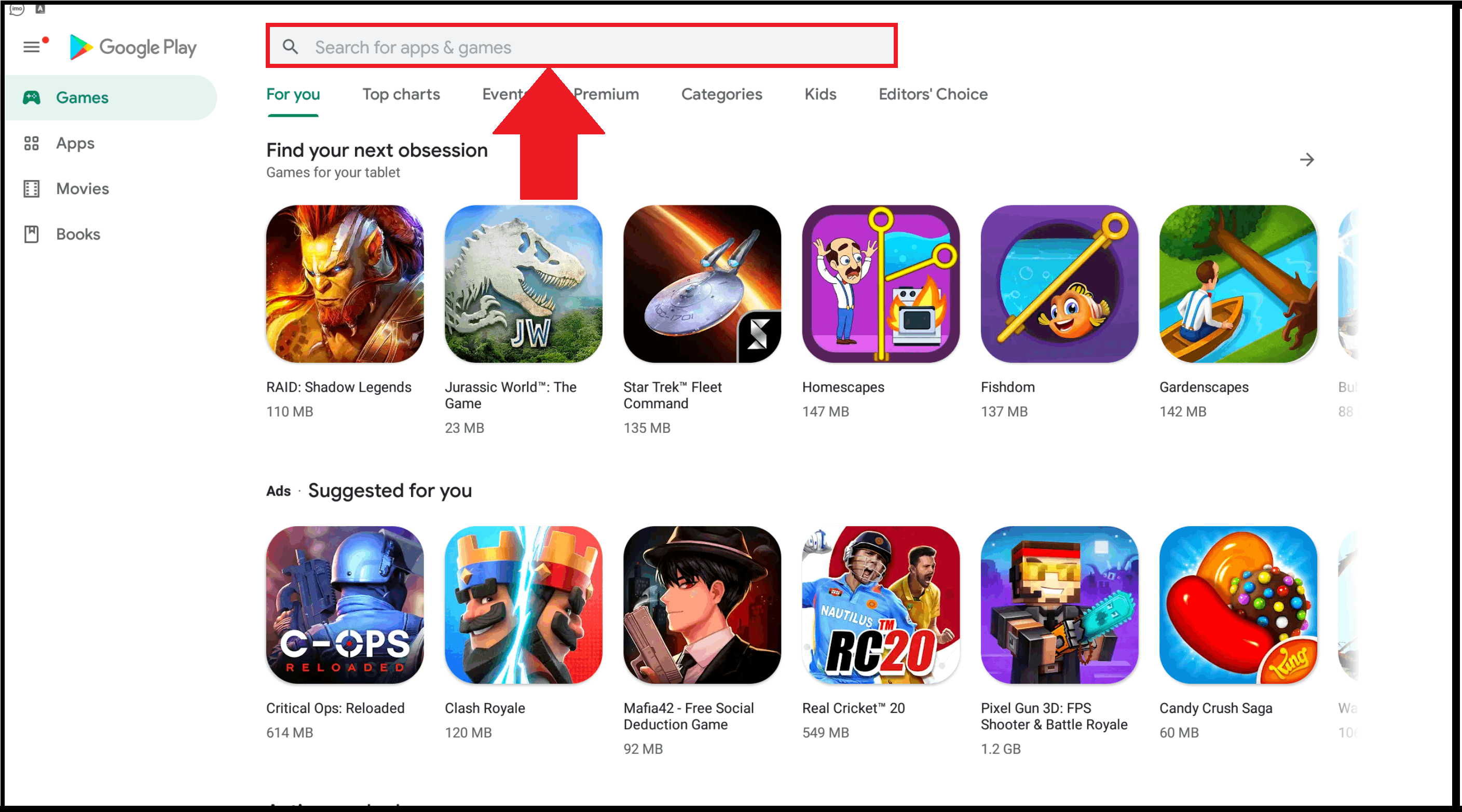The image displays the Google Play Store interface. Starting from the top, on the left is a hamburger menu icon with a red dot indicator, next to which is the Google Play logo. Adjacent to the logo is a search bar featuring a gray background, a magnifying glass icon, and the placeholder text "Search for apps & games" in faint gray. This search bar is emphasized with a bright red rectangle and a large red arrow pointing towards it.

Below the Google Play icon, there is a row of category icons: a video game controller, four dots in a square pattern, a film clapperboard, and a book. These icons correspond to the categories: Games, Apps, Movies, and Books respectively.

Next, a green underlined "For you" section is visible, followed by other categories such as Top charts, Events (partially obscured by the red arrow), Premium, Categories, Kids, and Editors' Choice. 

Beneath these categories, black text reads "Find your next obsession - Games for your tablet" followed by a series of game icons including Raid: Shadow Legends, Jurassic World: The Game, Star Trek Fleet Command, Homescapes, Fishdom, and Gardenscapes.

Further down, an advertisement banner titled "Just for you" features various game suggestions with their logos and icons. These suggested games include Critical Ops: Reloaded, Clash Royale, Mafia 42: Free Social Deduction Game, Real Cricket 20, Pixel Gun 3D: FPS Shooter & Battle Royale, and Candy Crush Saga.